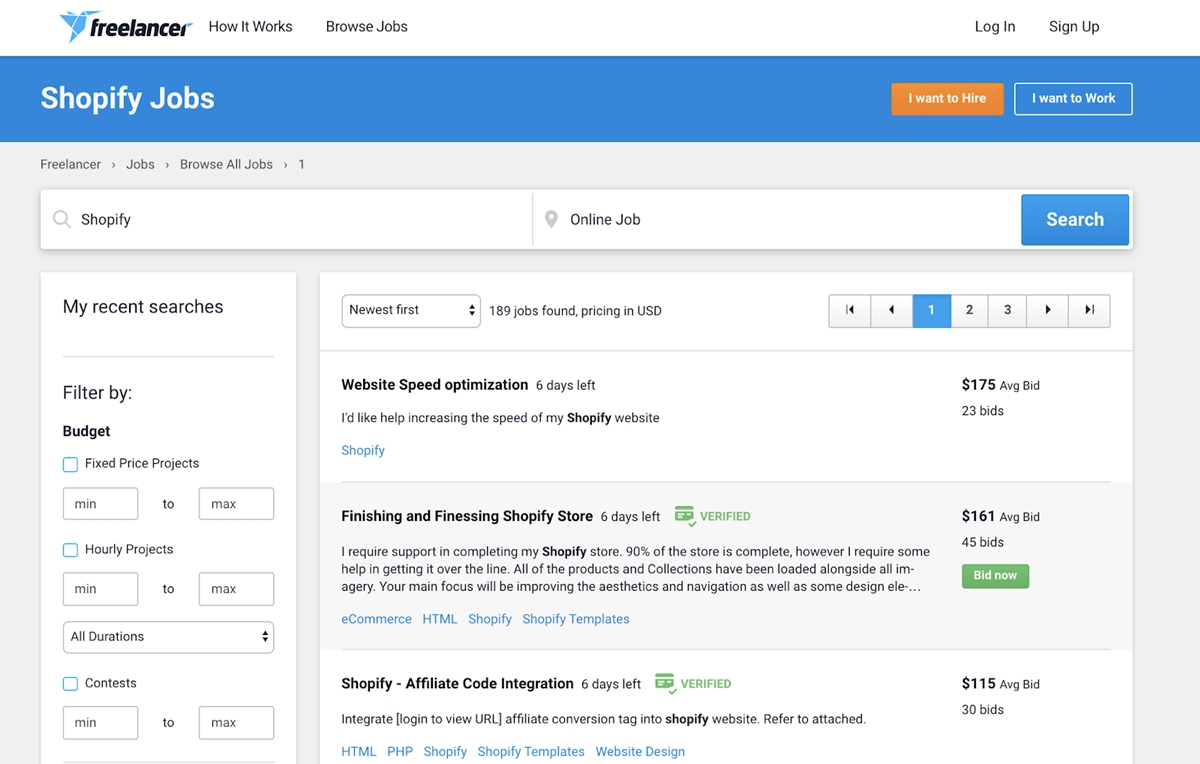The image depicts a screenshot from a freelancing website featuring a bird logo prominently at the top, symbolizing the freelance platform's brand. Adjacent to the logo, there are two primary navigation links: "How It Works" and "Browse Jobs." On the top-right corner, there are buttons for "Login" and "Sign Up," facilitating user access and registration.

Centered at the top of the page, a search query for "Shopify" has been entered, and above the search results, it lists "Shopify jobs" alongside two actionable buttons: "I want to hire" and "I want to work." Below this, the search interface is detailed with the location setting marked as "online job" and a prominent blue "Search" button.

The search results reveal that 189 jobs match the "Shopify" query, with three example listings displayed: "Website Speed Optimization," "Finishing and Finessing Shopify Store," and "Shopify Affiliate Code Integration." On the left-hand side, the sidebar includes sections for "Recent Searches" (currently empty) and various filter options like budget, project type (fixed price or hourly), and project durations.

The screenshot comprehensively showcases the platform's interface and its robust job search capabilities tailored for Shopify-related freelance opportunities.